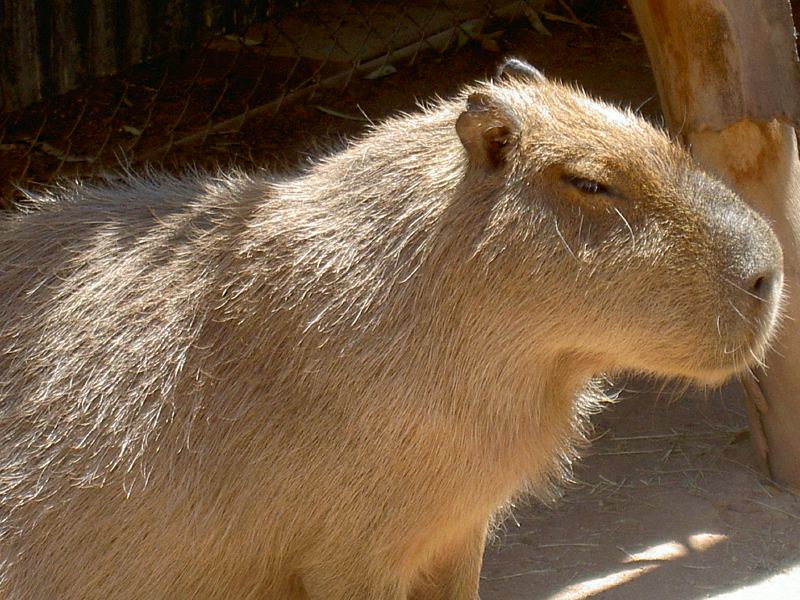In this image, we see a pale brown capybara positioned centrally in an outdoor setting, bathed in sunlight with a mixture of tan and darker brown fur, particularly around its ears and eyes, and a slightly blacker tone near its nose. The ground beneath is hard-packed dirt scattered with bits of grass and hay. Surrounding the animal, from the top left, there's a gate beside a corrugated metal wall, hinting at an enclosure likely within a zoo. Toward the upper right, a wooden stick or post extends downward to the middle right, with additional sections of the same dirt ground visible at the bottom right. The capybara, with its docile demeanor, short ears, large nose, and eyes situated on the side of its head, suggests a calm, non-aggressive nature.